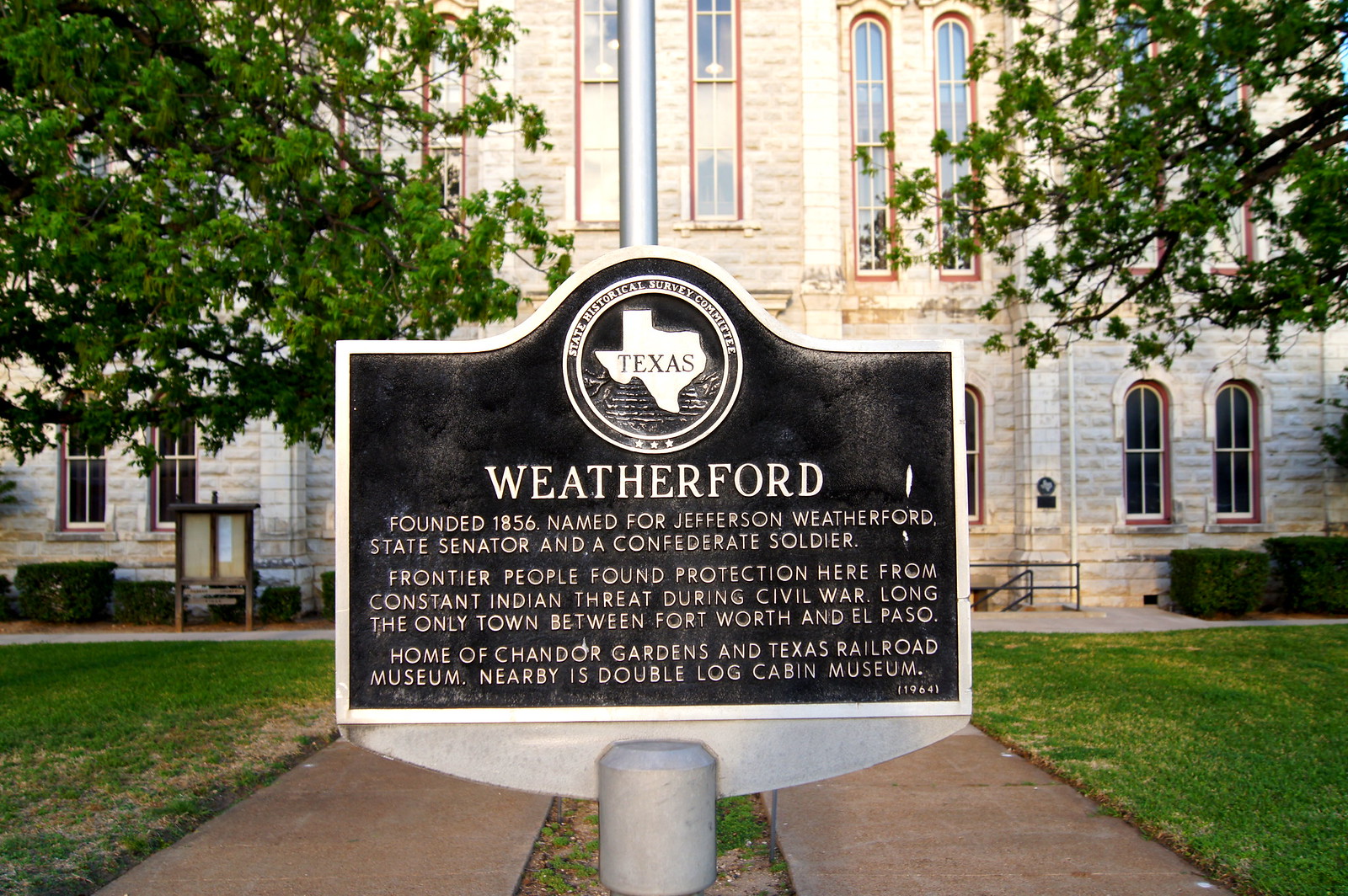The image features an outdoor scene dominated by a large black metal sign with white lettering. The sign has a silver frame and is mounted on a substantial metal base situated in a dirt area. At the top of the sign is a circular seal depicting the state of Texas, surrounded by the words "State Historical Survey Committee." The main text on the sign reads "Weatherford" in large white letters. Below that, in smaller white text, it details: "Founded 1856, named for Jefferson Weatherford, state senator and a Confederate soldier. Frontier people found protection here from constant Indian threat during the Civil War. Long, the only town between Fort Worth and El Paso. Home of Chander Gardens and Texas Railroad Museum. Nearby is Double Log Cabin Museum."

The sign stands in front of a large beige stone building with numerous arched windows. Two parallel walkways run from the foreground towards the back of the image, positioned behind the sign. Surrounding the building and walkways are patches of grass and some shrubbery. Additionally, branches and leaves from trees frame the upper portion of the image, adding a natural element to the scene.